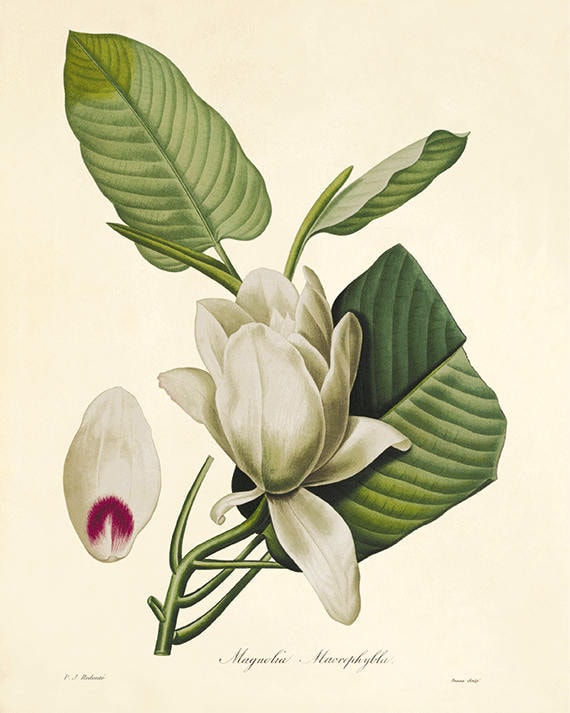The image depicts an artist's rendering of a magnolia flower on a vertically oriented, rectangular background that transitions from a pale peach to ivory. The detailed artwork showcases a magnolia flower with white petals, one of which is illustrated separately, revealing its oval shape and delicate purple-pink tint at the base. The flower includes three green leaves: one large leaf extending to the right with prominent veins, a smaller leaf rising beside it, and another leaf extending toward the left with a pointed tip. The magnolia bloom is partially closed, concealing the center. At the bottom of the image, a handwritten-style font identifies the flower as "Magnolia," followed by a dot and a blurred scientific name. The composition captures the elegance of the magnolia, highlighted by the varying hues of the background and the fine details of the petals and leaves.